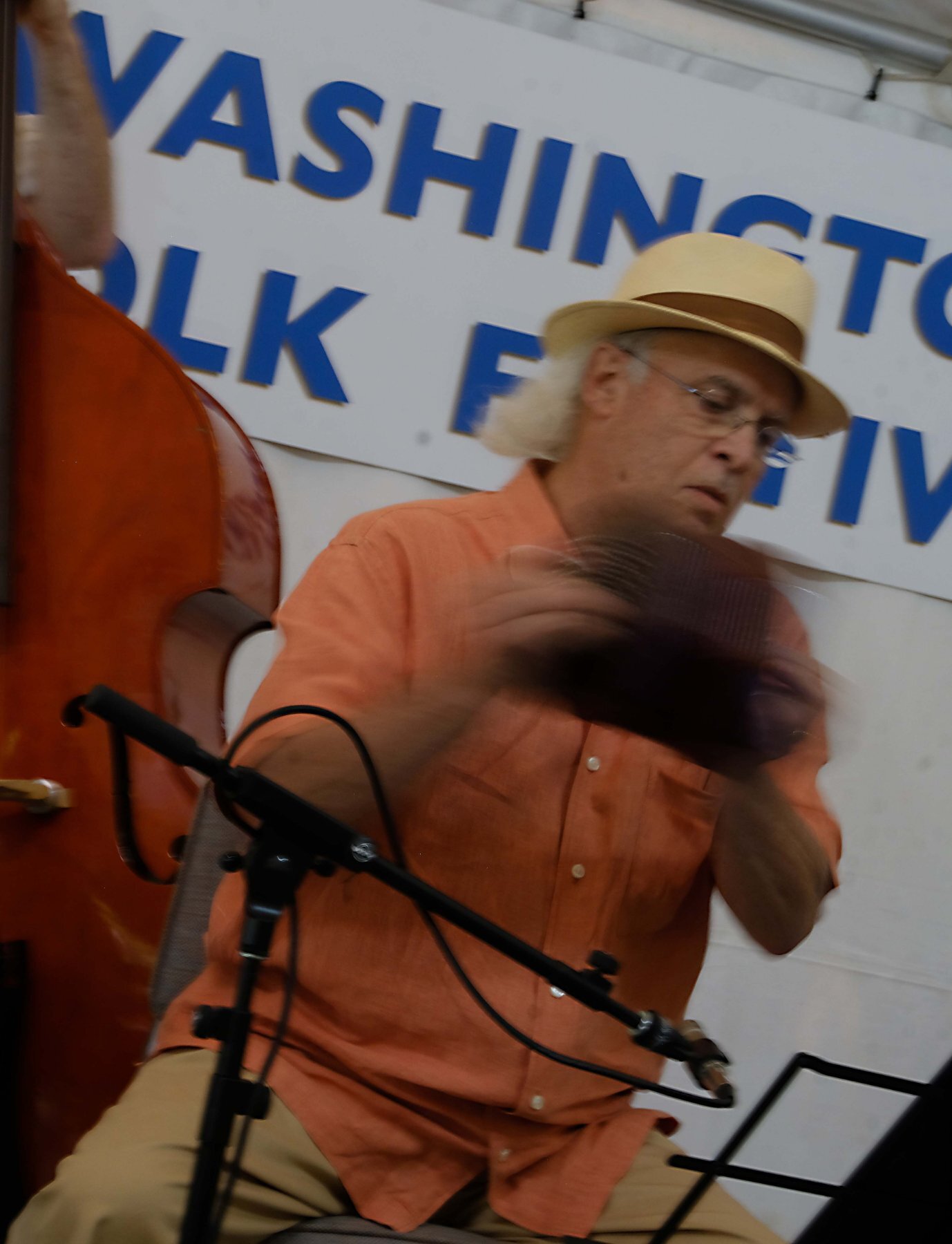The image captures an older man in the midst of a musical performance, suggesting a lively and engaging atmosphere typical of a folk festival. Center stage, the man is seated and wearing a distinctive tan hat with a dark band around the base, complemented by wire-rimmed glasses. His attire includes a salmon-colored, short-sleeved, button-up shirt with white buttons and a pocket on the left side, paired with tan khaki pants.

In front of him stands a microphone on a stand, angled towards his mouth, indicating he may be singing or about to address the audience. He grips an instrument with both hands that appears blurry in the photo due to its rapid movement, suggesting it could be a shaker or a small, fast-moving accordion-like instrument. To his left, a large stringed instrument, likely an upright bass or cello, is partially visible with an arm extending from the top left corner, playing it.

The backdrop features a white banner with blue horizontal lettering that partially reads "Washington Folk Festival," reinforcing the setting as a folk music event. The overall imagery, including his dynamic posture and the surrounding musical elements, paints a vivid picture of a spirited and authentic folk performance.